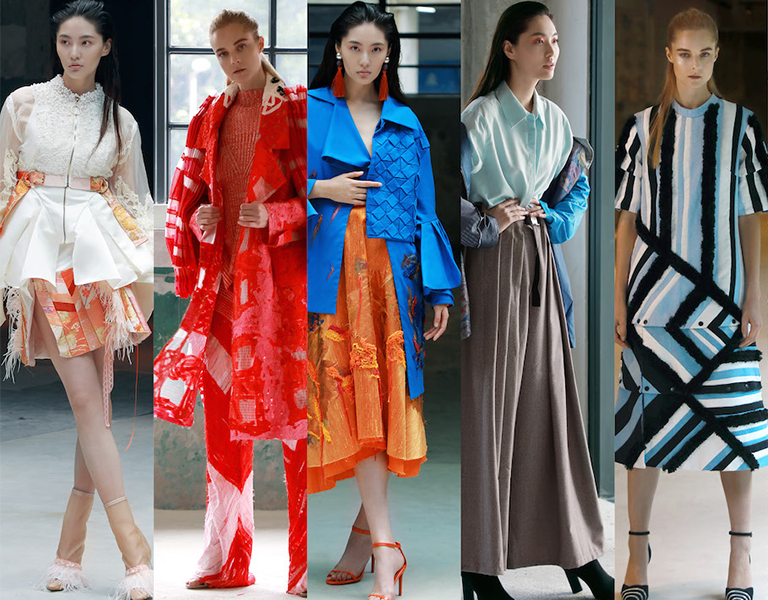This is a composite image showing five different models, each wearing avant-garde fashion ensembles at a fashion show. The models are a mix of Asian and Caucasian women, each presenting distinct and eclectic styles.

Starting from the left, the first model, who appears Asian with black hair, is dressed in a white top paired with an orange patterned skirt that features intricate strings hanging down. She completes her look with feathered boots.

The second model to the right is showcasing an elaborate ensemble of red and white hues; she wears an orange robe over matching pants and a red sweater. Her hair, a reddish-brown shade, is pulled back elegantly.

The central model captures attention with her bold accessories – long red tasseled earrings – and a striking outfit consisting of a misshaped blue jacket, an orange skirt, and orange high heels.

The fourth model is dressed in a more subdued combination of a light blue shirt and a gray skirt. Over her elbows drapes a blue jacket, and she has black shoes to match. She also appears to have black, straight hair.

Finally, on the far right, the model with dirty blonde hair is attired in a multidimensional dress with blue, black, and white stripes intersecting in varying directions. Her look is completed with black high heels.

Each outfit is uniquely layered and textured, displaying a mix of modern and asymmetrical designs that are both striking and unconventional.